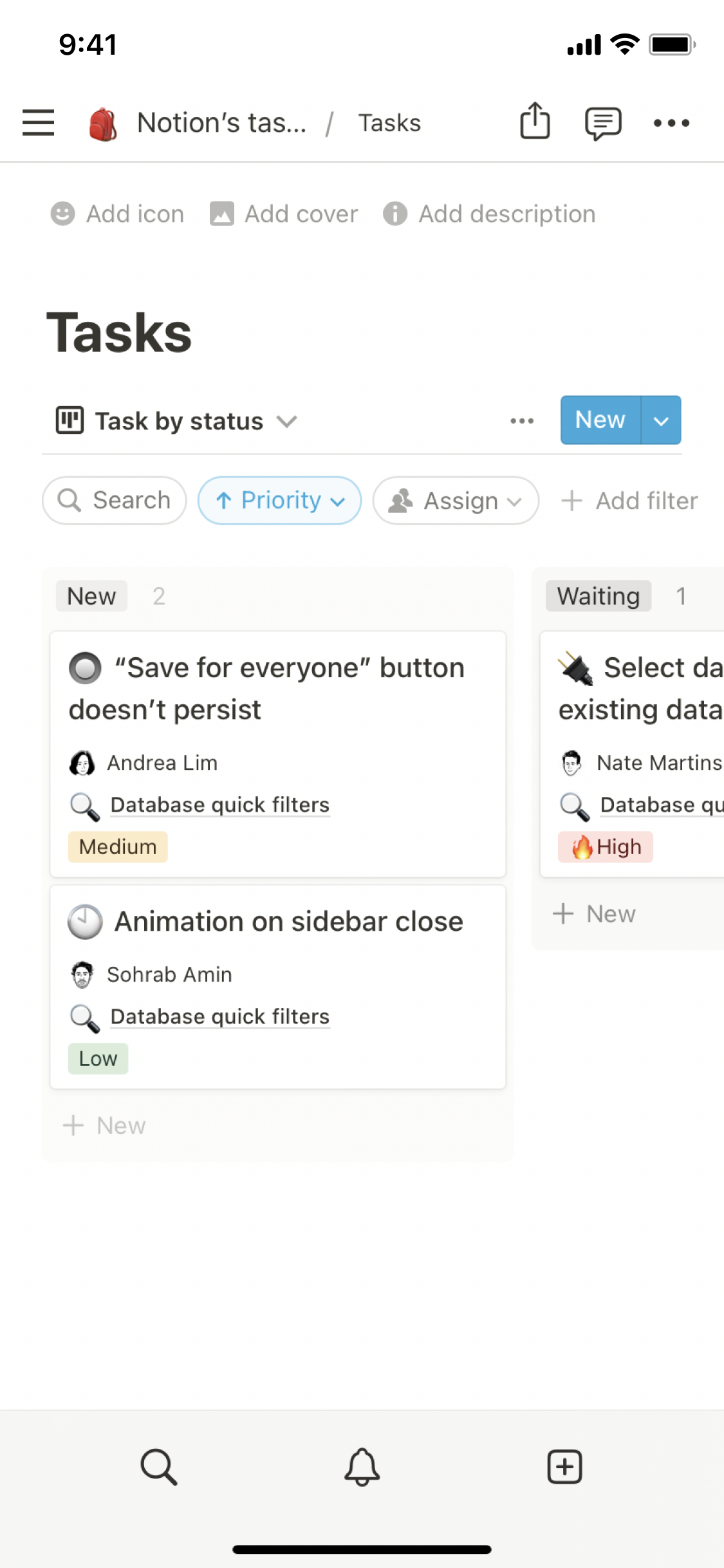This image is a screenshot from a mobile device displaying a task management app interface. The background is predominantly white, offering a clean and light appearance. The status bar at the top indicates a fully charged battery, strong Wi-Fi reception, and full cell signal. The time displayed is 9:41.

In the upper left corner of the app interface, there is a hamburger menu icon, which allows access to additional menu settings. Next to it, the text "Notions Tasks" is visible, indicating that the user is operating under the name Notion. Adjacent to this are two icons: a sharing icon resembling a square with an upward-pointing arrow, typical of Apple iOS, and a messaging icon.

Below this header, the word "Tasks" is prominently displayed in bold text. The tasks are sorted by status, specifically by priority. The list includes several tasks with varying priority levels:

1. "Save for Everyone Button Doesn't Persist" by Andrea Lim, marked with medium priority and highlighted in yellow.
2. "Animation on Sidebar Closed" by Sohrab Amin, marked with low priority and highlighted in green.
3. An unreadable task by Nate Martins, marked with high priority indicated by a red color and a fire symbol next to it.

The detailed priority indicators and the inclusion of task assignees suggest a well-organized and functional task management system.